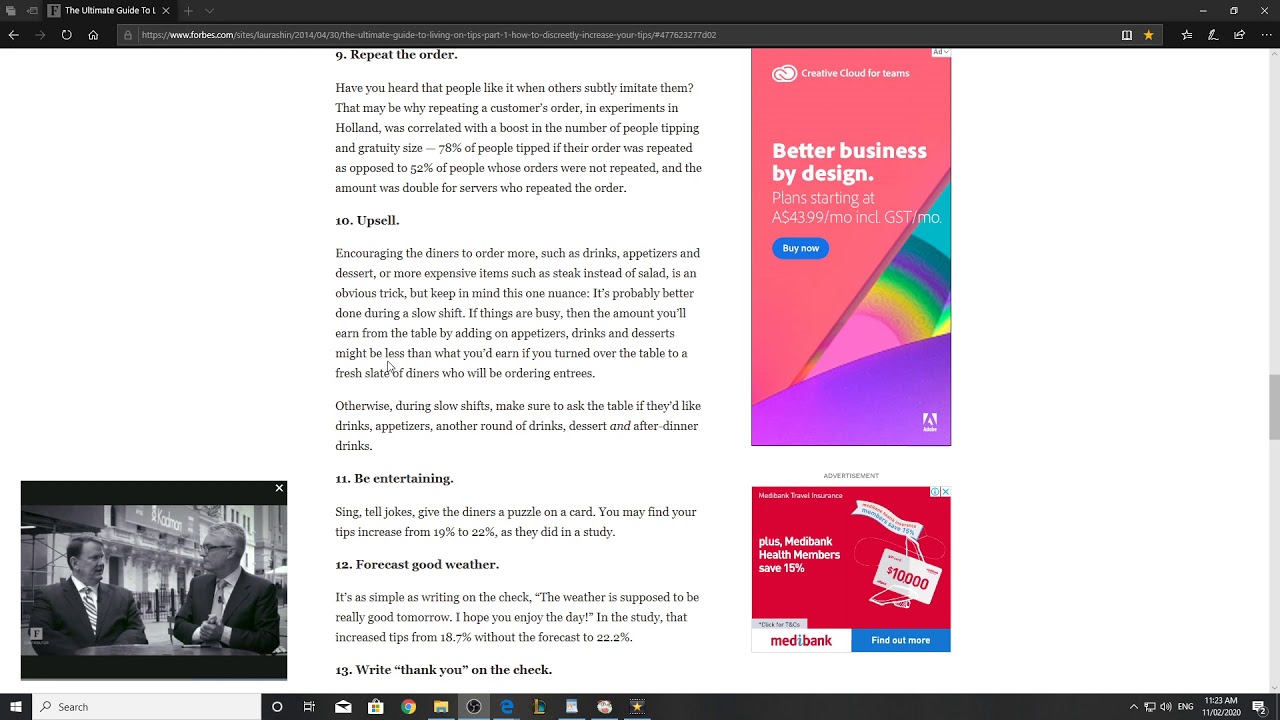In the upper left corner of the image, there is an open browser tab titled "The Ultimate Guide to Living on Tips - Part One: How to Discreetly Increase Your Tips" on Forbes.com. The URL in the search bar reads: https://www.forbes.com/sites/laurashine/2014/04/30/the-guide. 

Centrally located in the image is a tip highlighted as number nine, which states, "Repeat the Order." It explains that research from experiments in Holland indicates that subtly imitating customers by repeating their orders can boost gratuity sizes. Specifically, 78% of people tipped when their order was repeated, compared to 52% who did not tip when their orders were not repeated. Moreover, the tip suggests that doubling servers who repeated the order can be effective.

Tips numbered 10 through 13 are also visible, which include:
- 10. Upsell 
- 11. Be Entertaining
- 12. Forecast Good Weather
- 13. Write Thank You on the Check

In the bottom left corner, there is a photograph of two men seated at a table, seemingly engaged in conversation. On the right side of the image, there is an advertisement block that reads, "Better Business by Design Plan starting at $43.99."